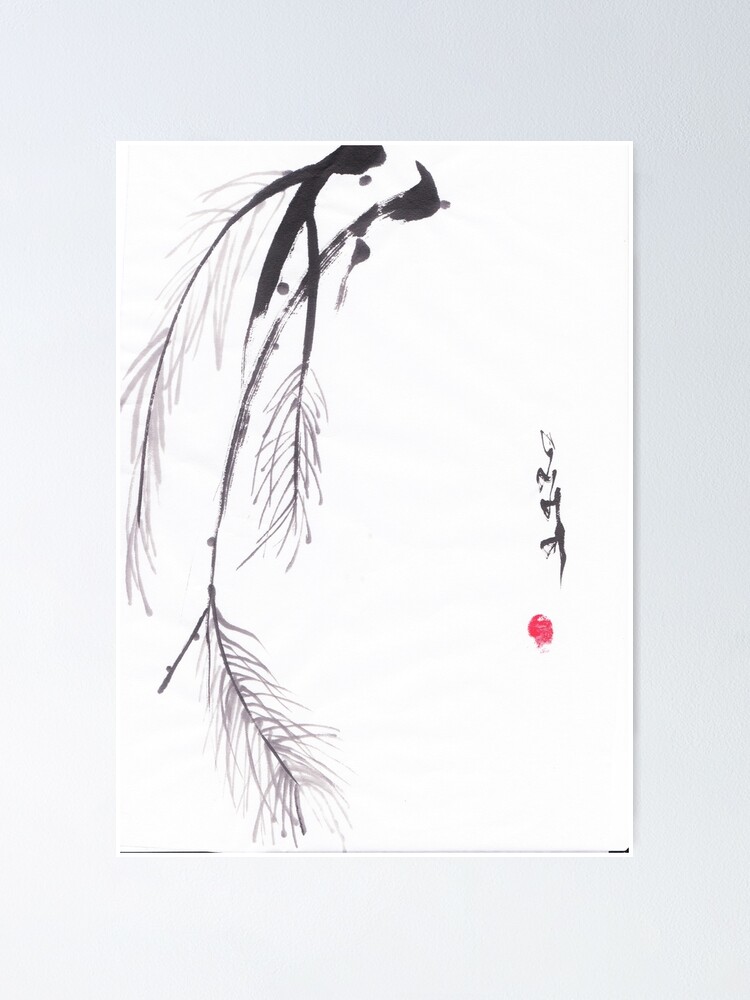This image features a minimalist, black-and-white painting on a white canvas that is mounted on a light blue wall. The painting primarily depicts three to four pine branches rendered in black ink, with variations in intensity from thick, dark strokes to lighter, more diluted ones. The branches originate from the top center and extend downwards mostly to the left side of the canvas, adorned with feathery needle-like leaves that are painted in finer, more delicate strokes, resembling pine needles or fern-like leaves. On the right side of the canvas, there are black squiggly lines that could be interpreted as text or abstract shapes, likely suggesting an Asian influence, possibly Japanese or Chinese. Below these lines, in the middle right of the canvas, is a distinctive red dot that resembles a thumbprint, contributing a splash of color to the otherwise monochromatic artwork. This subtle, intricate piece of art embodies characteristics of Sumi painting and exudes a serene, minimalist aesthetic.